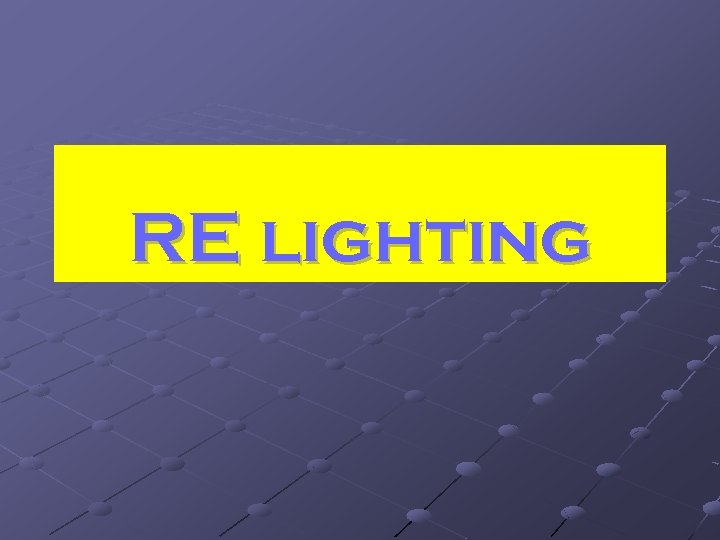The image features a striking, computer-generated background with a dark blue-purple flooring that stretches out into the distance, gradually becoming enveloped in a light purple fog. The floor is intricately designed with a grid-like or tile pattern, where each intersection point is marked by a gradient circle that transitions from dark purple to light purple. This background bears a resemblance to an inclined chain link fence viewed from a diagonal perspective, giving it a dynamic, fading effect. 

Dominating the center of the image is a bright yellow rectangular box that spans horizontally from left to right. Centered within the yellow rectangle, bold purple text reads "RE LIGHTING" in all capital letters. This vivid color contrast and detailed graphical design suggest that the image might be used as a header or a promotional display, potentially related to an electrical or lighting theme.